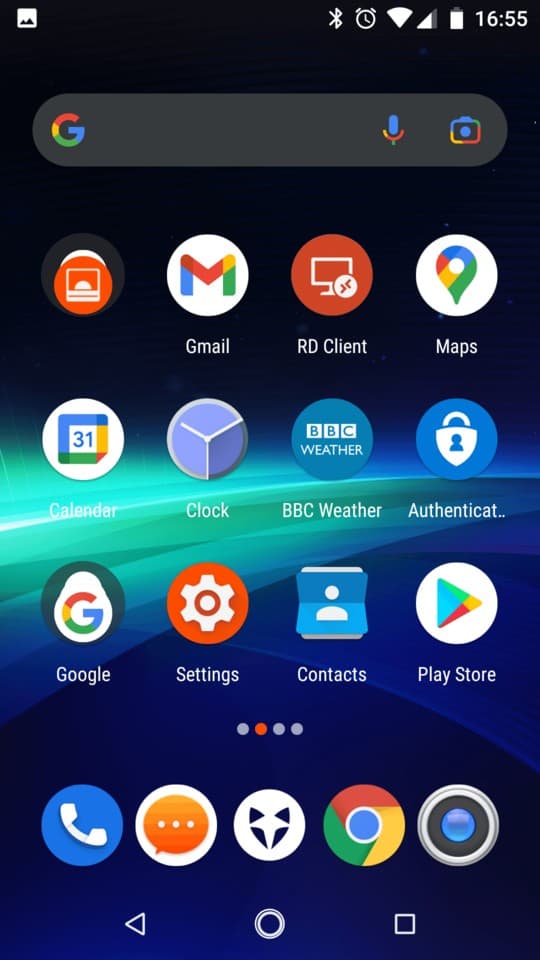Here is a detailed and cleaned-up caption for the image described:

---

This is an image of the home screen of an Android smartphone. The background features a colorful design with the top half in black and bluish lines forming a pattern in the middle. At the top of the screen, the notification bar displays various icons, including Bluetooth, alarm, Wi-Fi, phone signal, and the current time, which reads 16:55.

On the main page, just below the notification bar, is a Google search bar. Beneath that, there are three rows of app icons, each row containing four apps. The first row includes one app without a name, Gmail, RD Client, and Maps. The second row features Calendar, Clock, BBC Weather, and Authenticator apps. The third row includes Google Settings, Contacts, and Play Store.

Below these rows, four dots indicate the presence of multiple home screens, showing that this is the second screen. At the bottom of the screen, five app icons are displayed without names: the Phone app, Messages app, an unidentified app in the middle, Google Chrome, and the Camera app.

Finally, at the very bottom of the screen, there are three navigation buttons: Back, Home, and Recent Tabs.

---